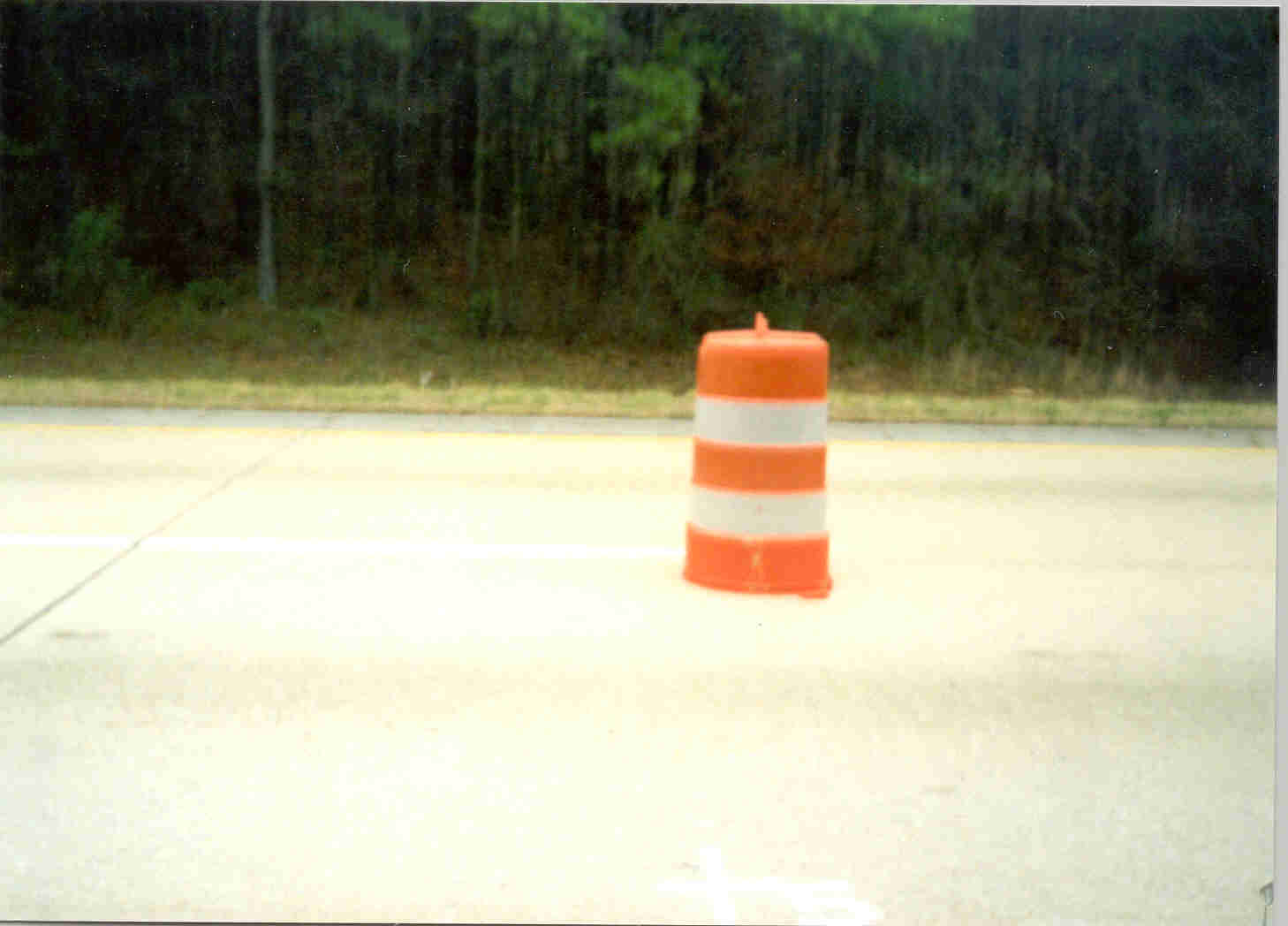This color photograph features a cylindrical object placed on the side of a road. The object, which resembles a traffic cone but with a more rounded top, is marked by alternating orange and white horizontal lines—three orange and two white. Of note, an orange line at the top includes a small protrusion in the center. The object is slightly wider at the base than at the top.

It is positioned on a yellow-painted pavement, which appears slightly out of focus, with a distinct white line running through it. A thin black line is visible at the bottom left edge, though its origin—whether part of the photograph or an external element—remains uncertain.

In the background, beyond the cylindrical object, a thin yellow line can be seen, followed by a narrow strip of grass. Tall trees with slender trunks and a mix of green leaves and darker foliage extend upwards, creating a dense, forested backdrop. The combination of elements suggests a semi-rural setting, possibly near a roadside clearing or park.